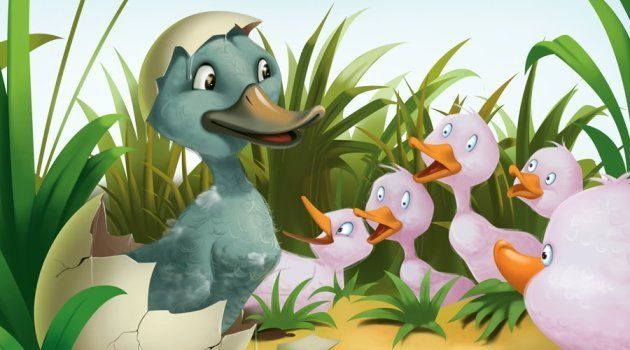In this charming cartoon illustration, a large, newly hatched blue duck with a brownish-blue beak and a fragment of its white eggshell perched atop its head stands proudly on orange dirt amidst a lush, green field under a clear, light blue sky. The blue duck, detailed with expressive white eyes and big black pupils, appears to be smiling warmly, almost as if introducing itself. It stands out dramatically from the five smaller, pink baby ducks surrounding it in shock and amazement, their wide, beady eyes and tiny black pupils conveying their disbelief. The pink ducks, each with orange beaks, are nestled in the green grass and appear to be nearly identical, emphasizing the unique appearance of their newly hatched blue companion.